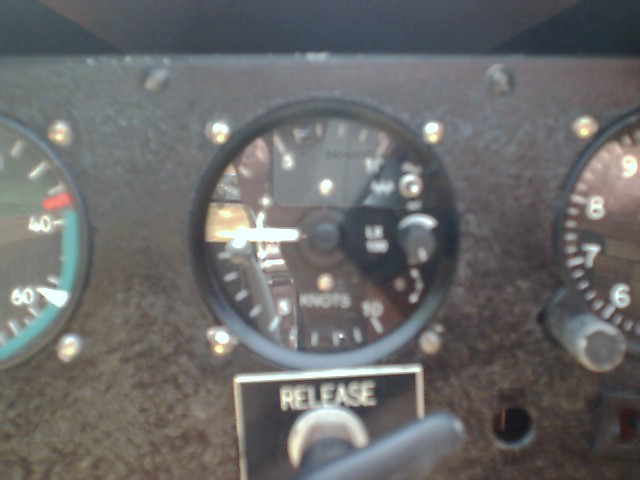A detailed dashboard, possibly from a boat, is depicted in the image. The dashboard has a gray background and features a series of gauges and indicators. At the bottom of the dashboard is a black handle labeled "RELEASE" in silver text. Surrounding this handle are several screws, securing the components in place.

On the left side of the dashboard, there is a gauge that measures from 1 to 8, though the left edge of this gauge is partially cut off in the view. The center of the dashboard prominently displays a large circular gauge that measures speed in knots, with markers at 0, 5, and 10 knots. The white indicator on this gauge points to 60, although it's unclear what specific measurement this relates to without more context.

The right side of the dashboard features another gauge that measures from 6 to 9, but like the left gauge, its right edge is also cut off. Above these gauges, there appears to be another section of the dashboard with additional controls, though it is not fully visible. A small hole is present in the bottom right corner of the dashboard, possibly for a purpose such as additional mounting or wiring.

Overall, the dashboard is characterized by its functional design, with clear indicators and sturdy construction suitable for marine environments.